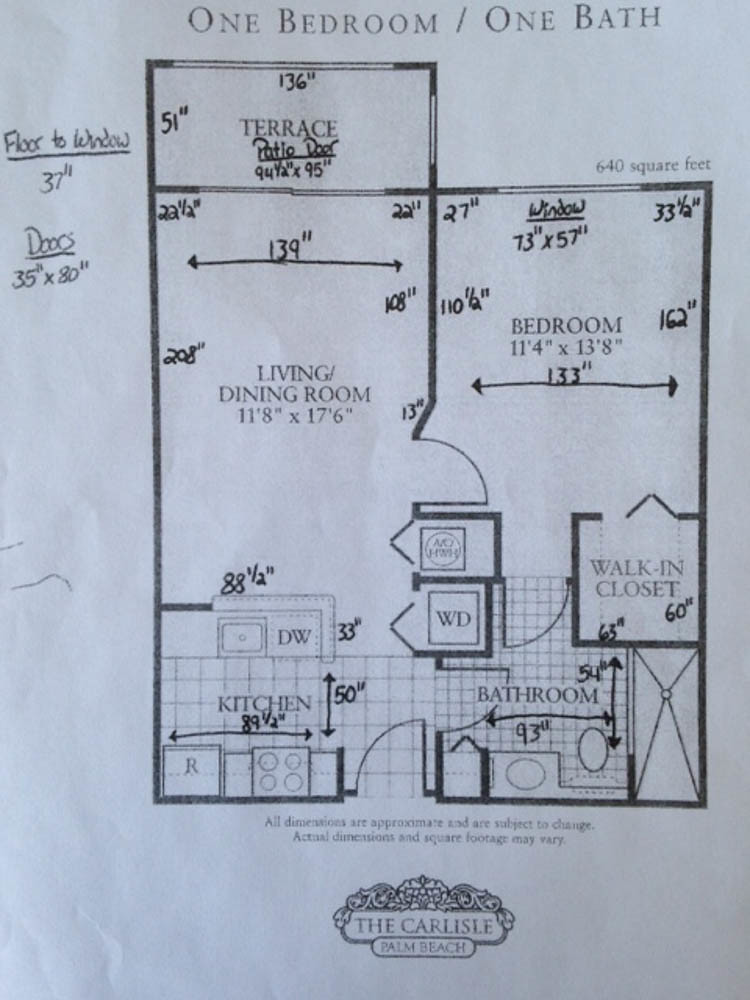A detailed annotated diagram of a one-bedroom, one-bath apartment interior. The diagram includes comprehensive dimensions of the entire living space. Instead of showing just the overall measurements, each individual wall in the living room, as well as the sizes of the windows and doors, are meticulously annotated. It seems designed for a project requiring precise square footage of walls. The layout features a living room (11 by 17.6 feet), a small kitchen, a walk-in closet, a washer-dryer unit, a water heater, a bathroom with a shower, and a terrace. The entire apartment covers 640 square feet. Annotations, including specific room dimensions and double-arrow markers indicating distances, cover the diagram. The drawing corresponds to an apartment in "The Carlisle" located in Palm Beach.